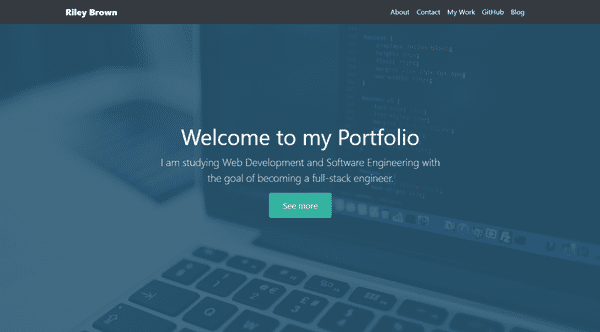The image is a color screenshot showcasing Riley Brown's portfolio website in landscape format. At the top of the screen, there is a dark blue, almost black banner, with the name "Riley Brown" prominently displayed in white text on the left, using capital letters for both initials. On the top right of the banner, there are several navigation tabs labeled "About," "Contact," "My Work," "GitHub," and "Blog."

The background features a slightly dimmed, generic photo of a laptop screen and keyboard, providing a tech-oriented ambiance to the website. Overlaid on this background is the prominent white text "Welcome to my portfolio." Beneath this welcome message, in a smaller white font, it states, "I am studying web development and software engineering with the goal of becoming a full stack engineer."

Finally, a green button with white text reading "See More" is positioned below the introductory text, inviting viewers to explore further.